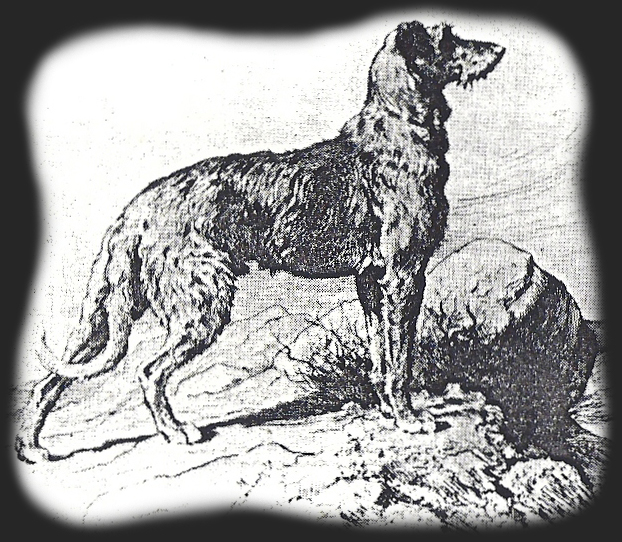This black and white drawing depicts a side view of a dog standing on a rocky cliff or hill. The dog, a medium-sized, muscular but not emaciated animal, is looking intently to the right. It has shaggy, short fur that appears messy and matted in various directions. Three of its legs are straight while one leg is slightly raised backward. Its tail curves downward and then upward. In front of the dog is a prominent rock, with smaller rocks and some vegetation nearby. The ground seems barren, resembling dirt. Surrounding the image is a wavy black border, adding a unique frame to the artwork, which gives an antique or vintage feel to the overall presentation.